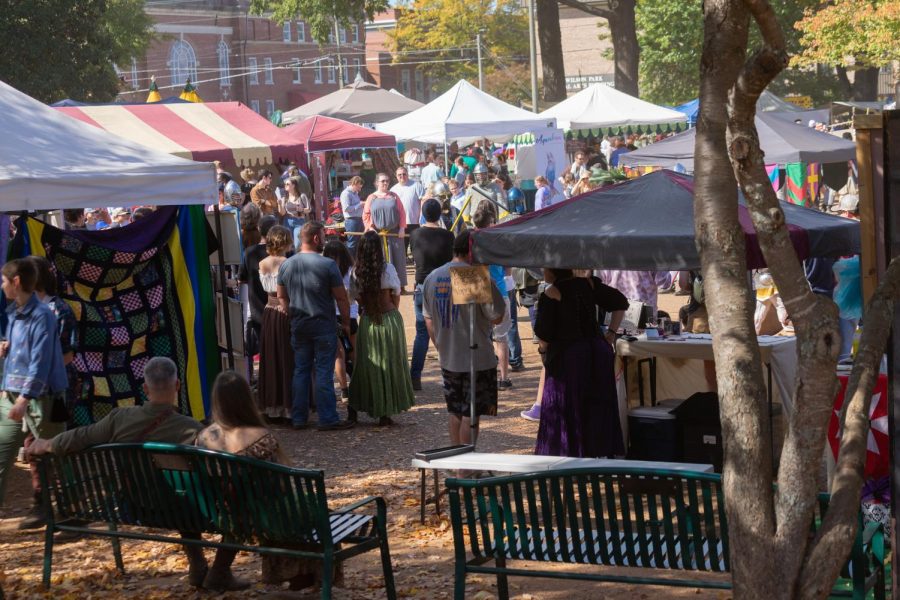The photograph captures a vibrant renaissance festival set in a town square, bustling with activity. The central area features a crowd gathered around men in knight uniforms and silver helmets engaging in a lively jousting or sword-fighting display. Women in renaissance attire, characterized by long skirts, leather belts or vests, and white peasant blouses, complement the historic atmosphere. The scene is framed by numerous canvas-topped booths, each with distinct fabric roofs—some striped red and white, others solid red or plain white—housing various craftspeople selling their wares. 

On the left, a colorful crocheted afghan with a blue, yellow, and checkerboard pattern hangs in display. Nearby, a green metal park bench hosts a couple engrossed in the festival's activities. Predominantly visible are the backs of spectators, most of whom are dressed in period-appropriate clothing, indicative of a European influence with embroidered off-the-shoulder tops and full skirts. 

The festival takes place under clear skies with sunlight brightening the crowd. A picturesque backdrop includes tall brick buildings and power lines, enhancing the quaint charm. To the right, a tree with brown bark provides natural framing, while green metal park benches stand in the foreground, contributing to the scene's communal and festive ambiance.